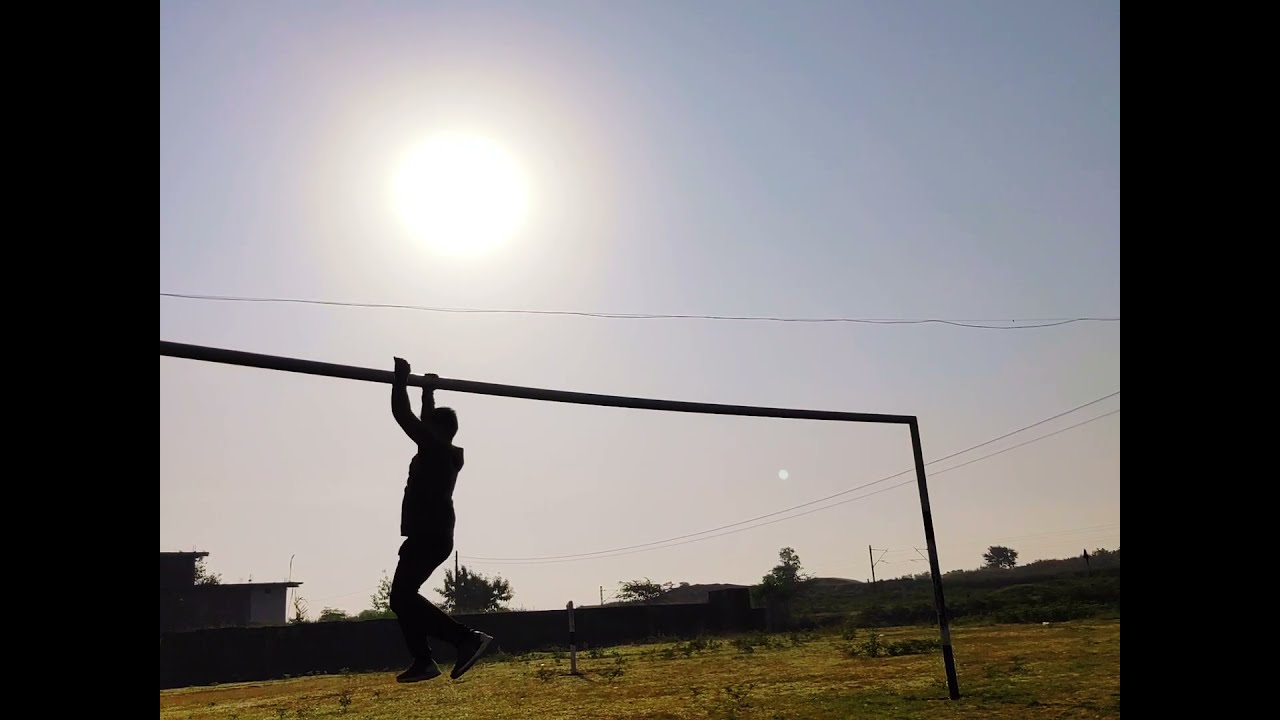The image depicts a vast, flat landscape bathed in daylight with a clear, light blue sky. The sun is prominently shining near the center, creating a hazy backdrop. In the foreground, there is a grassy field or park area with sparse vegetation, including a few tiny trees and a row of shrubs. Dominating the left side is a large fence and a rectangular building that appears to have two stories, possibly a shed. Further in the distance, a series of power lines stretch across the horizon. Central to the image is the silhouette of a man hanging from a horizontal pole elevated above the ground, seemingly pulling himself across. The scene is framed by black borders on both the left and right sides, giving the impression of columns, which adds an immersive or cinematic touch to the composition.